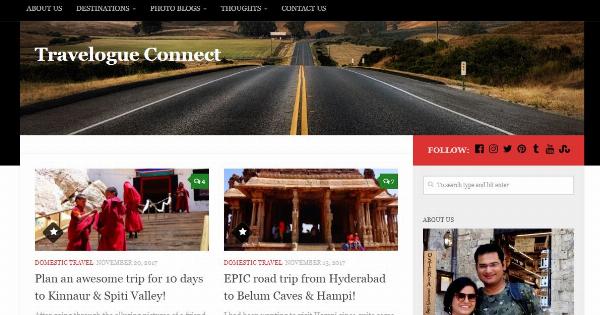The webpage for Travelog Connect prominently features an image of a picturesque two-lane road with solid yellow stripes down the middle, framed by expansive fields and scattered trees typical of farmland countryside. The road inclines slightly downhill, curves to the right, and eventually vanishes into the distance, evoking the open road’s allure. On the top left side of this image, in white letters, is the title "Travelog Connect," accompanied by a red banner urging visitors to follow the site on various social media platforms like Facebook, Instagram, Twitter, Pinterest, and YouTube.

Below the main image, the page includes linked articles with accompanying photos. One advertisement entices visitors with a 10-day trip to Kanar and Spiti Valley, featuring an image of three individuals in red robes standing on a tall staircase leading into a building. Adjacent to it, another advertisement promotes an epic road trip from Hyderabad to Belum Caves in Hampi, illustrated with a photo of a temple-like structure with wooden pillars and an open interior.

Further down on the right side is an "About Us" section displaying a photo of the founders, a man and a woman, both with dark hair—he wears glasses and she sports sunglasses—posing in front of a white stone building. This organized layout emphasizes travel destinations and provides a personal connection with the site's creators.